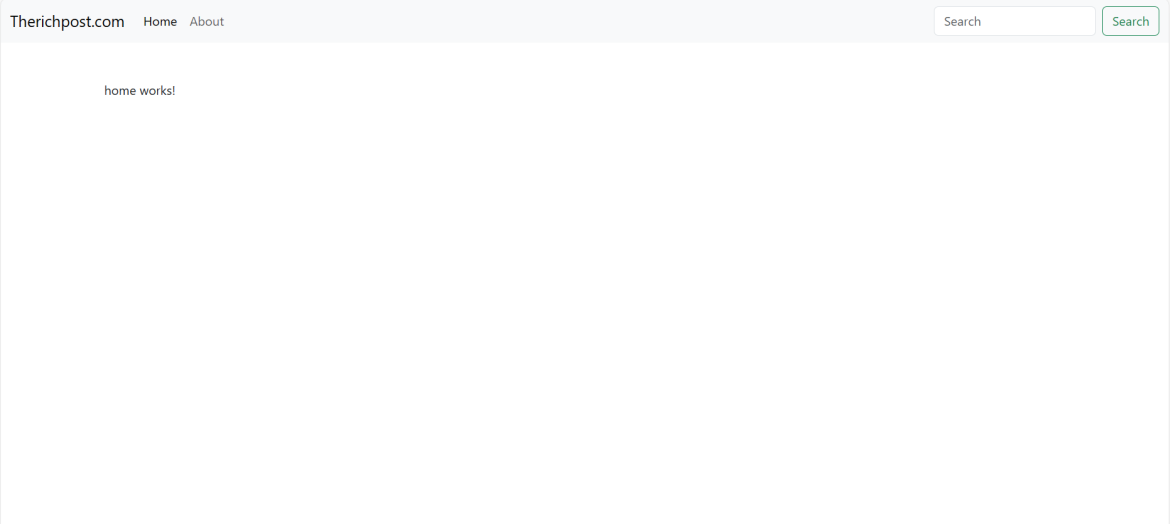Here's the revised caption:

"This partial screenshot captures the top half of a chart with a very light gray header. The header includes the text 'therichpost.com' on the top left, followed by 'Home' and 'About' immediately to the right. On the far right, there is a search bar accompanied by a search button outlined in green. The main window of the screenshot is predominantly white with only two prominently displayed words in black lowercase text: 'home works!' The phrase 'home works' is presented as two separate words with an exclamation point following 'works.' The box containing the text has a gray border that matches the color of the header. The bottom section of the chart is not visible in the screenshot."